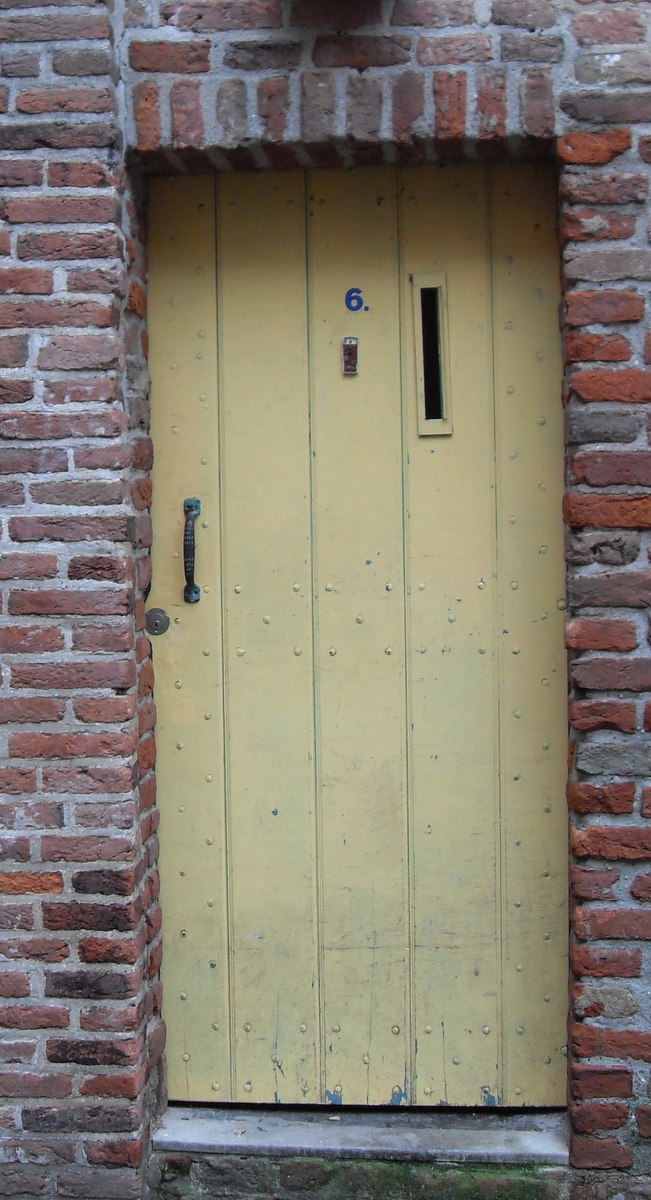This is a color photograph taken outdoors during the daytime, showcasing a distinct and detailed doorway built into the side of a red brick building. The door is set into the brickwork, with a small ledge at the bottom requiring a step down to exit. Made from vertically placed wooden planks, the door is painted a dull yellow-golden hue. A blue number 6 is positioned modestly above a peephole to the left. The door also features a narrow vertical slit window on the top right side. A black, U-shaped handle with a circular lock beneath it is situated on the left. The brick facade surrounding the door is composed of varied red and grayish-red bricks, outlined with cement. The photograph captures the intricate details and textures of both the door and the brickwork, highlighting the craftsmanship of the entryway.